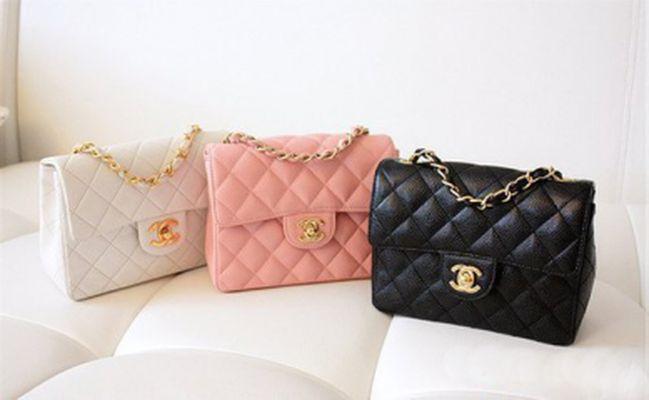This color photograph captures three elegantly displayed handbags, positioned side by side on a deeply padded, cream-colored surface which appears to be a couch or settee. The padding beneath the bags forms distinctive, fluffy-looking squares or deep curves, adding a plush texture to the scene. Each handbag features a diamond-shaped design with the iconic Chanel logo — two interlocking Cs, facing opposite directions — prominently displayed in the center. The bags are adorned with gold clasps and handles, giving them a luxurious appearance:

- The handbag on the left is white with a gold clasp and handle.
- The middle handbag is pink, also featuring a gold clasp and handle.
- The right handbag is black, maintaining the same gold detailing.

The background reveals a cream-colored wall, with a slender vertical strip of a light gray wall visible in the upper left corner, possibly indicating its edge, which might be that of a wall or window. This adds further context to the setting, enhancing the sophisticated ambiance of the image.